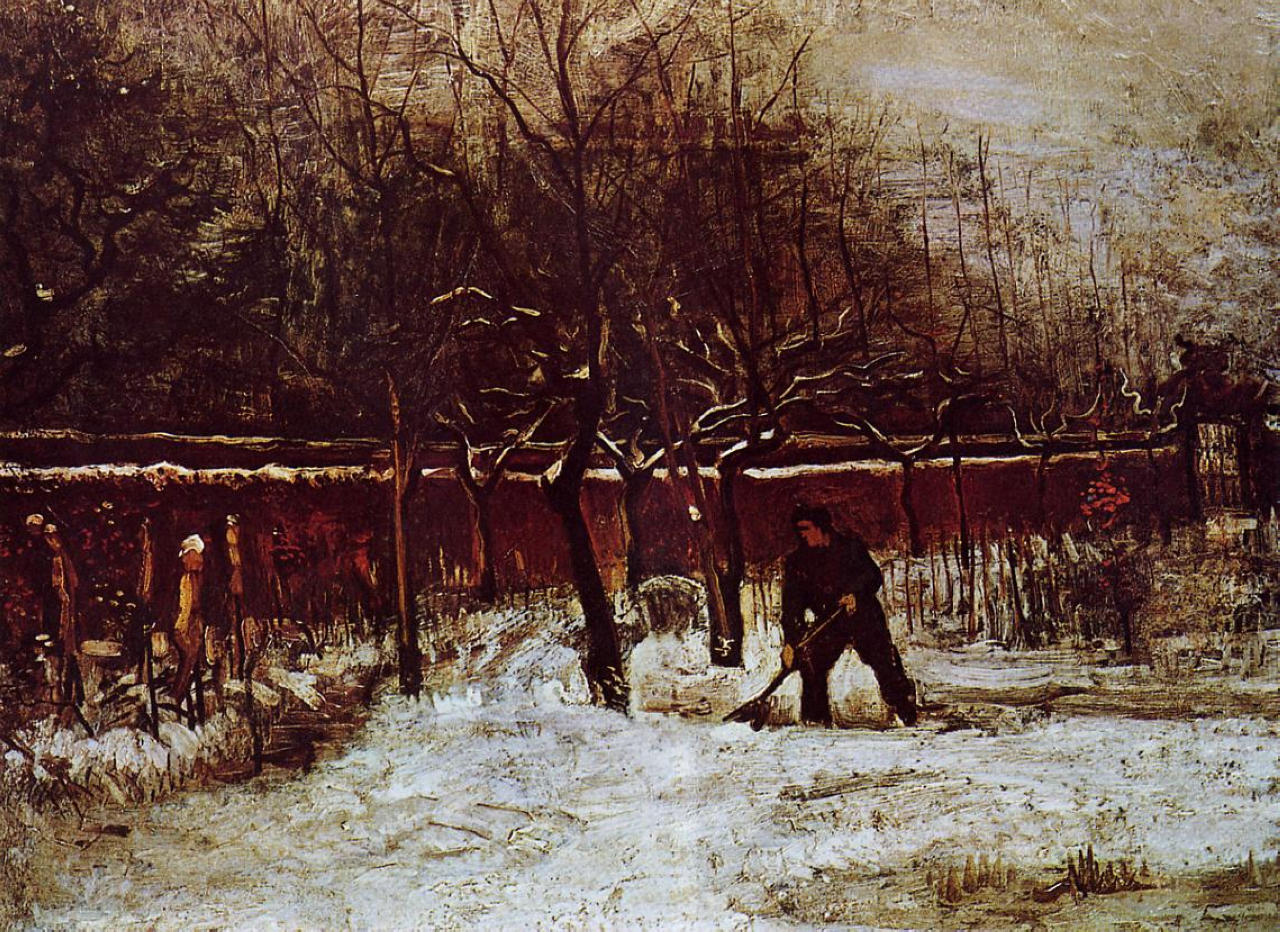The image is a painting depicting a somber, snowy outdoor scene dominated by muted and dark colors, primarily white, brown, and an orange-red hue. The central focus is a lone man positioned slightly to the right of the center, dressed in dark clothing with dark hair, engaged in shoveling snow, possibly with a shovel or a snow brush. The ground, mostly covered in snow, reveals patches of green and yellow, indicating mixed terrain or partially melted snow. Bare trees with brown trunks and snow-dusted branches frame the painting, particularly on the left and middle sections. A brown, murky stream snakes through the scene, adding to the overall gloomy atmosphere. Faintly, off to the left, there may be another figure amidst the trees, enhancing the sense of isolation. The sparse use of color, with brief pops of an orange-red, possibly from leaves or fruits on a tree or shrub, contrasts starkly against the predominantly white and brown landscape, contributing to the painting's melancholic mood.